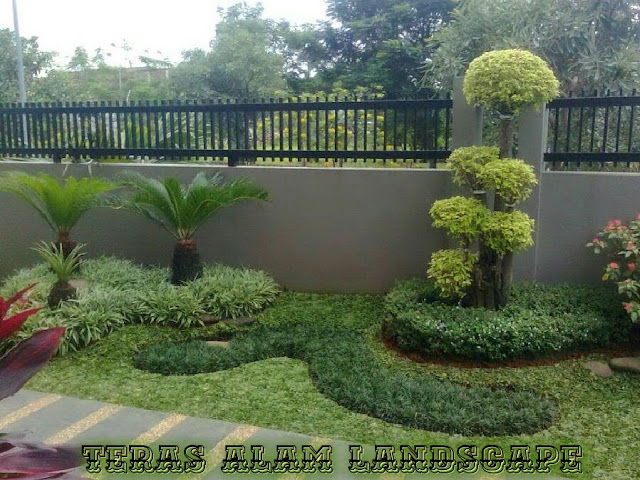The image depicts a meticulously designed garden landscape, likely used in a landscaping portfolio with the caption "Terra's Alam Landscape" at the bottom. The setting features a grey wall topped with a short black metal gate. In front of the wall, various plants and trees are arranged on green grass. On the left side, there are two fern plants with lighter green, long leaves below them. To the right, a taller plant, characterized by mushroom-like clumps of leaves, is surrounded by shorter bushes. There are also some red petals visible in the corner of the image. At the far back, beyond the wall, a dense arrangement of trees creates a lush background. The grass in the foreground exhibits a distinctive design with varying shades of green, separated by a sidewalk edged with blue stripes, suggesting a well-thought-out and artistic landscape layout.